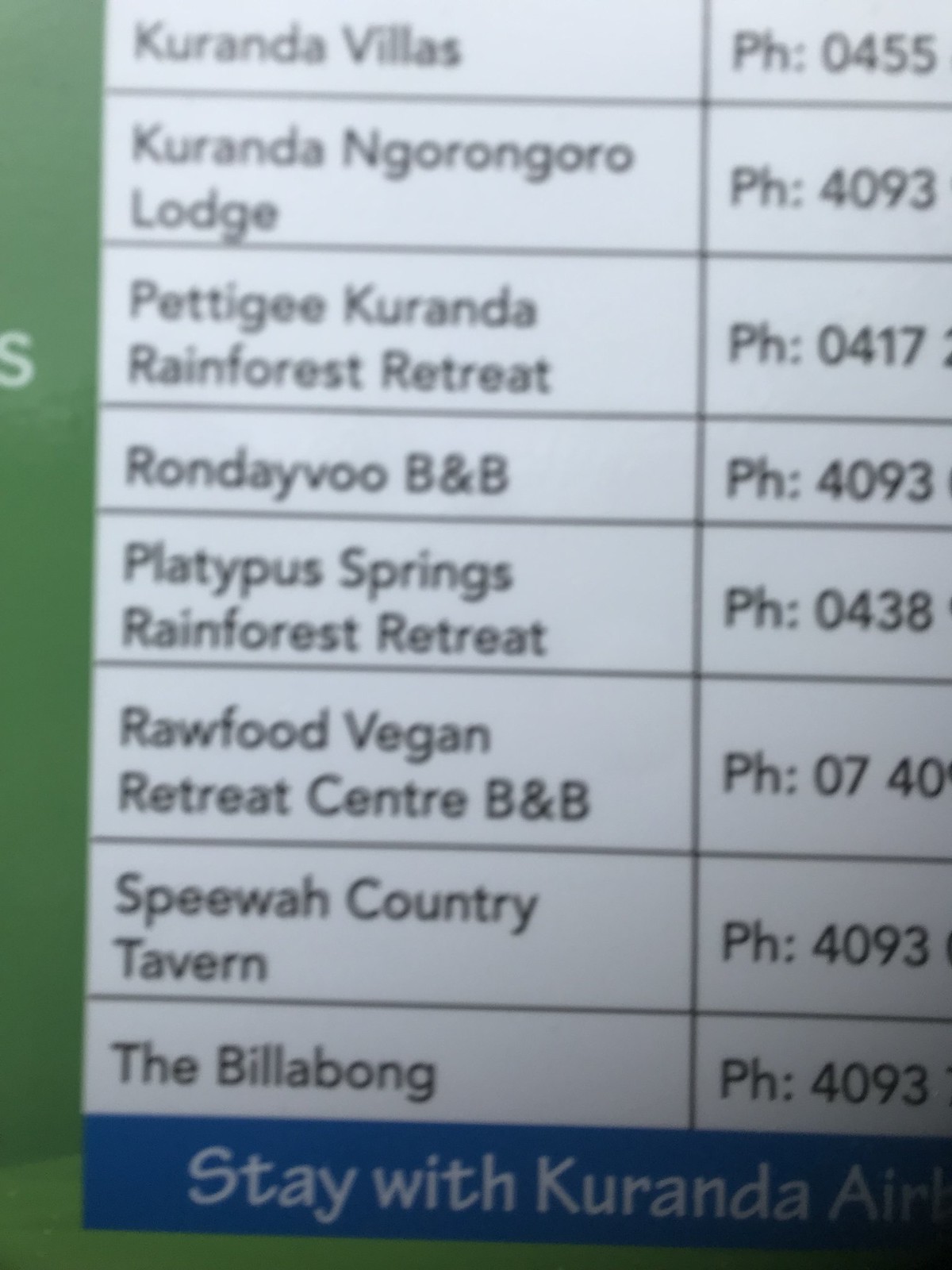This close-up color photograph captures a printed list, possibly from a website, featuring various accommodation options, likely in Australia. The image is defined by a green vertical border on the left with the letter "S," and a horizontal blue border at the bottom adorned with the phrase "Stay with Kuranda." The main content is presented on a white background in the form of a grid, organized into rows and columns. The left column details the accommodation names, each paired with partial phone numbers in the adjacent column. The listings include: 

1. Kuranda Villas, phone 0455
2. Kuranda Ngorongoro Lodge, phone 4093
3. Pedigree Kuranda Rainforest Retreat, phone 0417
4. Rendezvous B&B, phone 4093
5. Platypus Springs Rainforest Retreat, phone 0438
6. Raw Food Vegan Retreat Center B&B, phone 0740
7. Spiewa Country Tavern, phone 4093
8. The Billabong, phone 4093

The photograph hints at a slice of serene lodging options, highlighted by familiar Australian geography terms like "Platypus Springs" and "Billabong," reinforcing its likely origin.